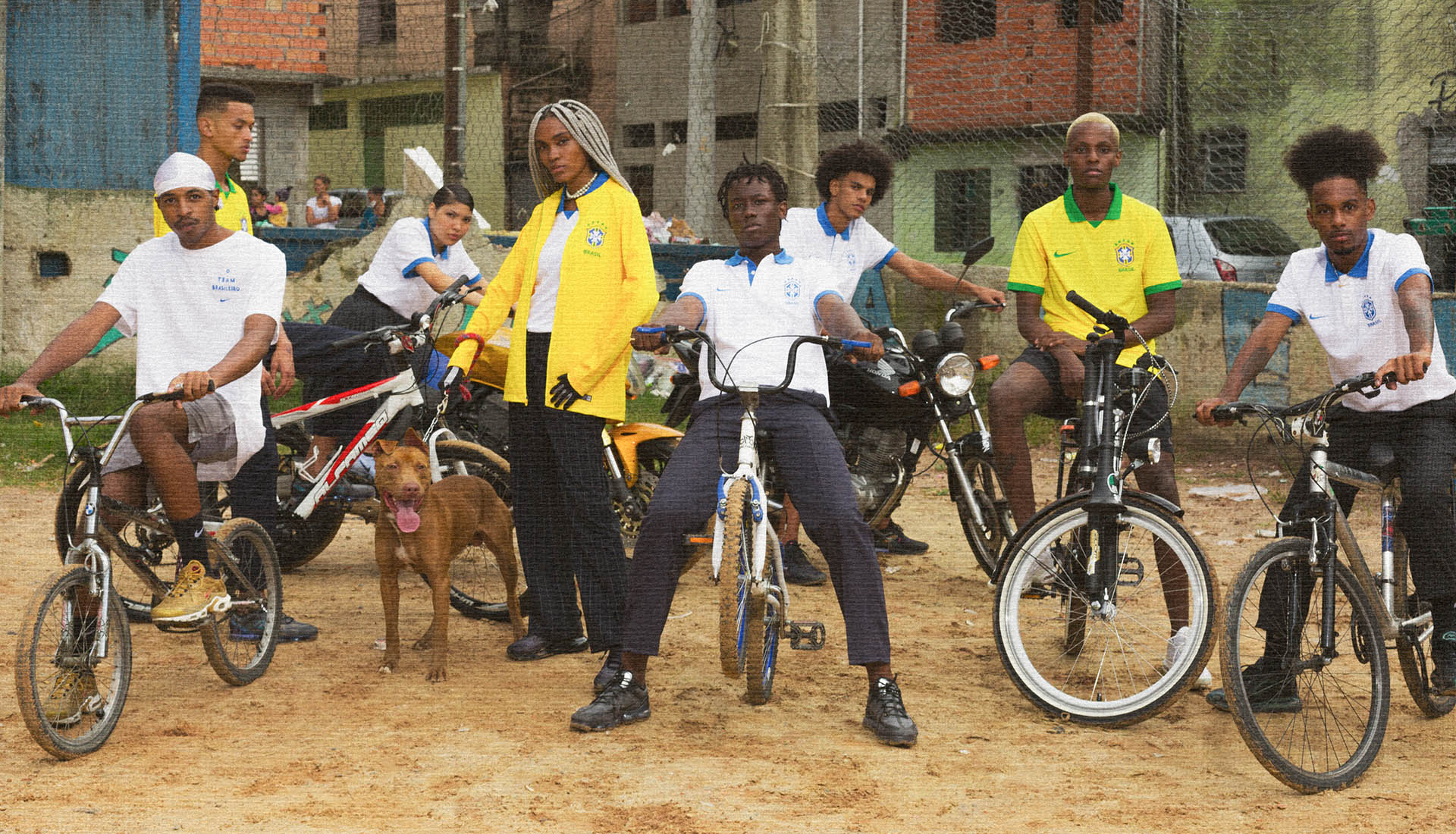In the photograph, a group of young people, looking like teenagers, are gathered in an alley, surrounded by buildings and a porch at the back. The scene feels somewhat staged, possibly for an advertisement or a music video. Everyone, except for one person, is on a bicycle. The exception is a slightly older woman who stands out as she holds a dog on a leash—it's not a friendly-looking dog, with its tongue hanging out menacingly. The group of individuals includes both girls and boys, who seem to be sporting very neat and clean attire, possibly school uniforms. Most of the young people wear white shirts with blue trim, while others don yellow shirts with green trim. The woman's jacket also shares the yellow and green color scheme, paired with a white shirt underneath and black pants. All the boys have on either black pants or dark shorts. They're all positioned horizontally across the image, with buildings and a porch where a couple of onlookers stand, observing the scene. The vibrant colors found in their clothing and surroundings include yellow, tan, beige, orange, green, brown, white, gray, silver, and blue, set against the backdrop of a Brazilian favela-like area.